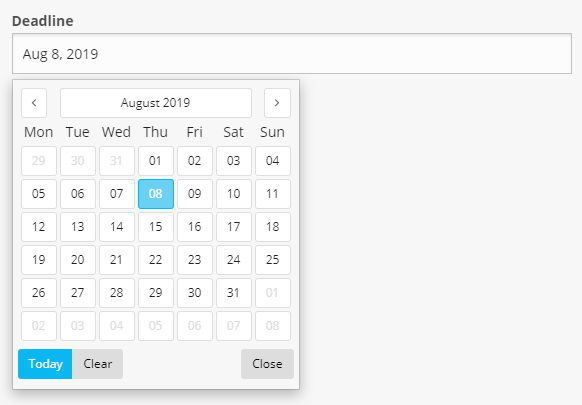This is a detailed and descriptive caption for the image provided:

"A cropped screenshot of a desktop calendar application is displayed. Set against a primarily gray background, the interface features very thin, sans-serif text indicative of a PC app rather than a mobile one. At the top left corner, the word 'Deadline' is prominently displayed in black text. Directly below is a text input bar with 'August 8th, 2019' typed in.

The primary focus of the screenshot is a calendar box towards the left, accentuated with subtle shadowing. The header within this box reads 'August 2019,' flanked by navigational arrows that allow month selection. The calendar grid begins with the last few days of July—29, 30, and 31—faded out to differentiate from the current month.

Each day of the week (Monday through Sunday) is aligned in columns, with notable emphasis on Thursday, the 1st, as the initial day of August that is fully visible. The current date, the 8th, is highlighted in blue with white text for easy identification.

Below the date grid, there are functional buttons: 'Today' in blue to jump to the present day, and 'Clear,' which when activated, deselects any chosen date. To the right, a grayed-out 'Close' button provides an option to exit the calendar view. This cropped image comprehensively captures the essential elements of the calendar interface."